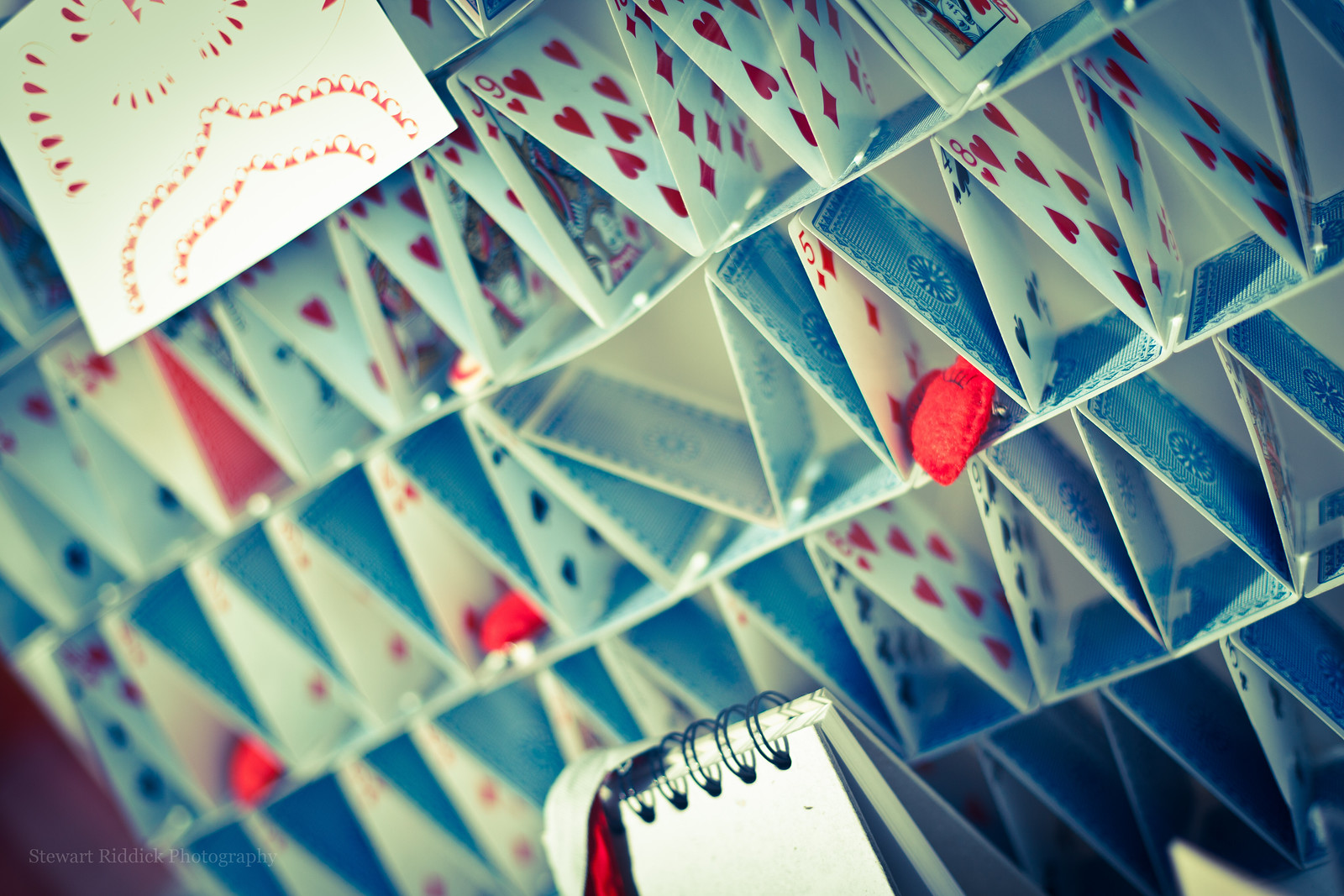This photograph captures a meticulously crafted house of cards, viewed from a 45-degree angle that tilts towards the right. The image is overlaid with a blue filter, giving the standard white playing cards a soft, pale blue hue. Each card features a simple blue design on the back, adorned with scalloped edges and a central medallion encircled by horizontal lines.

In the bottom center of the composition, there is a spiral notepad, flipped open to reveal its blank pages. The notepad is held together by five black spirals, providing a stark contrast against the blue-toned scene. At the bottom left corner of the photo, a watermark reads "Stuart Riddick Photography" in a subtle, transparent white font, marking the creative ownership of the image.